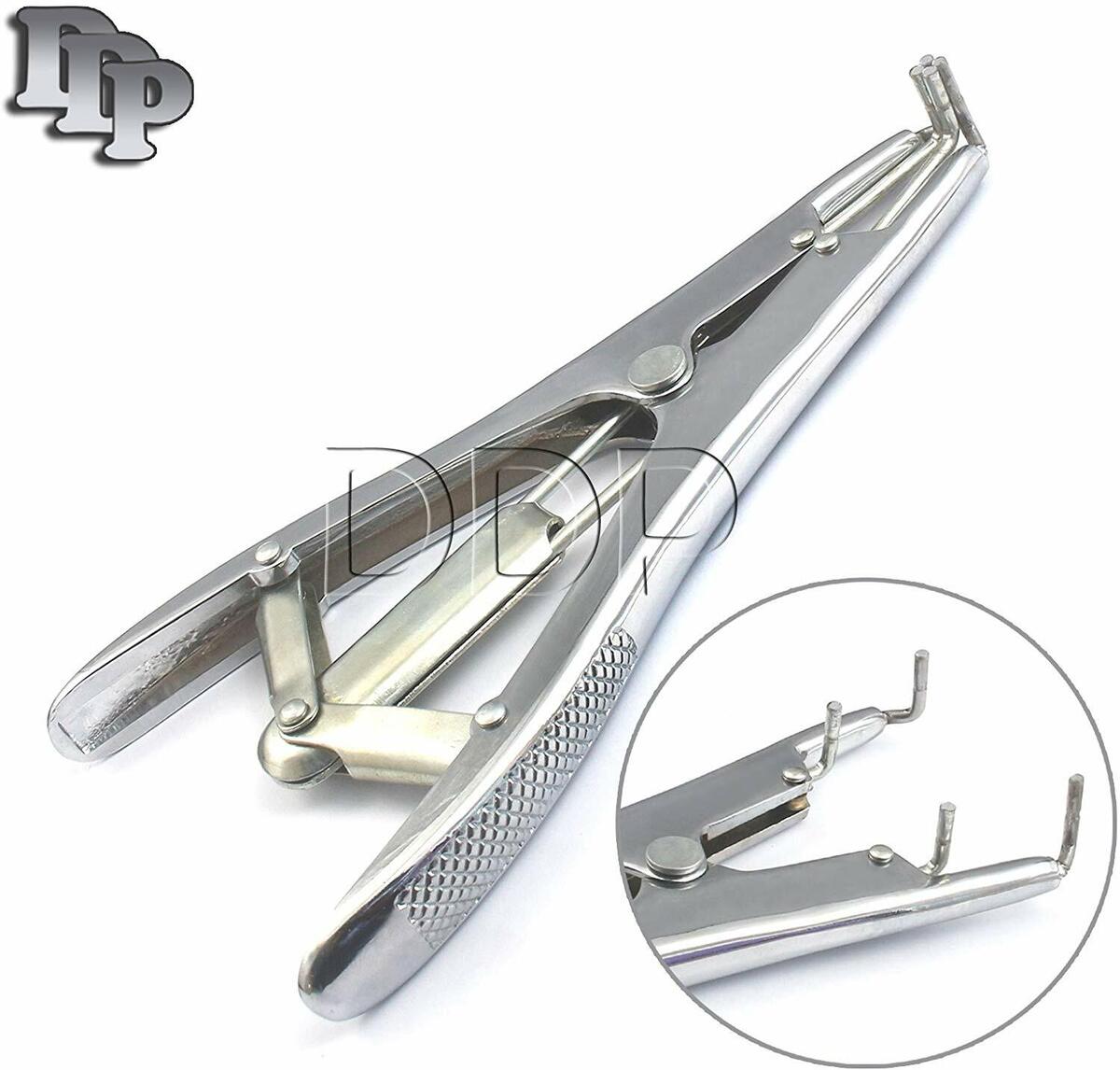The image depicts a silver metal tool set against a white background, prominently featuring the overlapping letters "DDP" in gray at the top left corner, likely representing a brand logo. The same "DDP" watermark can be seen in the center of the image, adding further branding identity. The tool itself bears two handles connected by a hinge and springs, suggesting it is designed to be held and operated with one hand. Squeezing the handles causes the top part of the instrument to open, revealing four small metal prongs. Additionally, a circular inset at the bottom right of the image provides a close-up view of the prongs in an open state, implying the tool's function is to grab or separate items. This tool appears to be specialized for use in automotive or mechanical tasks.